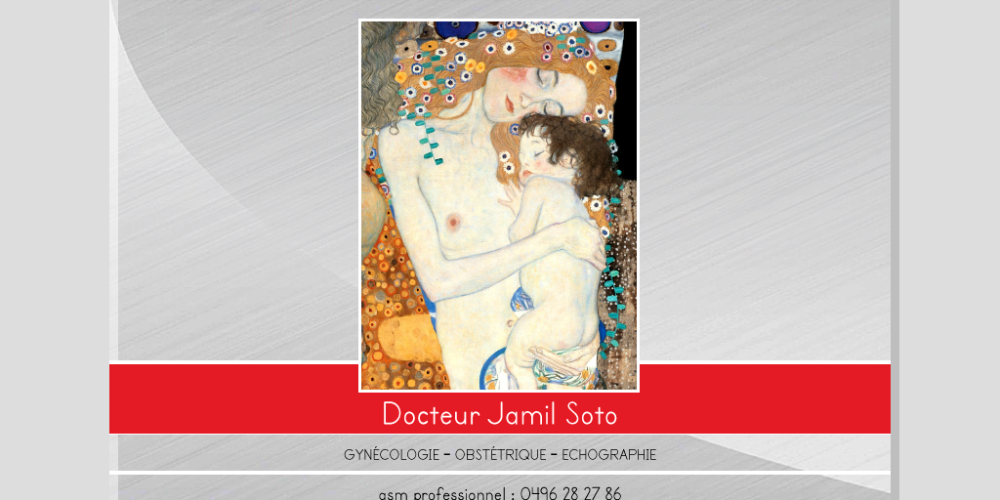An old-fashioned painting depicts a serene scene of a woman taking a nap, cradling her sleeping baby on her chest. The woman, with brownish blonde hair adorned with flowers in an array of colors—yellow, white, blue, pink, and red, interwoven with green vines—has her head gently resting on her baby's head in a tender embrace. Her right breast is exposed, while she holds the baby securely, who is only partially clothed with a blanket wrapped around his bottom. The baby, with dark brown hair, is nestled peacefully against his mother. The background is a mix of muted gray with shimmery streaks, complemented by brown and orange floral patterns and green vines. At the bottom, a red bar contains text that reads: "Dr. Jamil Soto, Gynecology, Obstetrics, Echograph, ASM Professional, 0496282786," suggesting this artwork is part of an advertisement for a gynecologist's office. The intricate details and mix of vibrant and soft colors add depth to the intimate moment captured in the image.